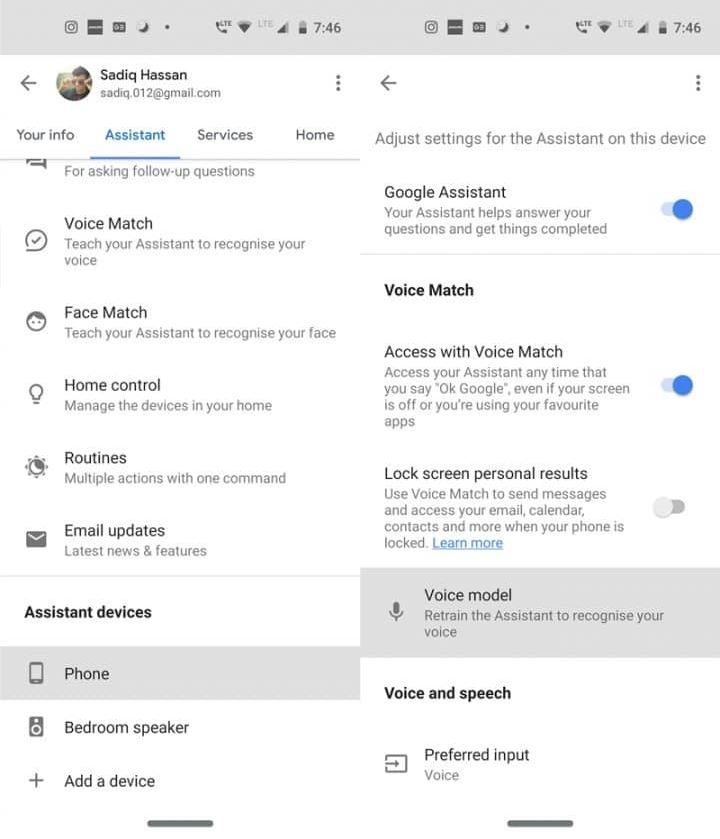This image consists of two adjacent screenshots, each framed with a white background and topped with a light grey banner. The images, which appear to be captures from a smartphone, display various user interface elements, including status bar icons indicating Wi-Fi signal, carrier name, battery level, and current time.

The left screenshot features a circular profile picture of Sadiq Hassan, accompanied by his name and email address. Below this profile section are navigation options labeled "Your info," "Assistant" (highlighted in blue, indicating the current view), "Services," and "Home." An arrow next to the profile picture allows the user to navigate back to a previous menu.

Further down in this screenshot are sections such as "Voice Match" for voice recognition training, "Face Match" for facial recognition training, "Home Control" (depicted by a light bulb icon) to manage smart home devices, "Routines" (represented by a sun and moon icon) for creating multiple actions under a single command, and "Email updates" for subscribing to news and features. Below these options, separated by a thin grey line, is a section titled "Assistant devices" on a white background, showcasing a phone icon labeled "Phone," a speaker icon labeled "Bedroom Speaker," and an option to add more devices.

The right screenshot, similarly styled, includes navigation and menu options at the top with a back arrow to return to the previous screen and three dots for additional settings. It prominently displays the header "Google Assistant," followed by a toggle switch marked "On" next to a description of the assistant's capabilities. A thin grey line divides this section from the "Voice Match" header.

Under "Voice Match," there are two toggled-on options: "Access with Voice Match" and "Lock screen personal results," each outlined in bold. The access setting allows the assistant to activate upon hearing "Okay Google," even with the screen off or when using apps, while the lock screen setting permits voice commands to interact with personal data such as messages, email, and contacts. A linked "Learn more" option provides additional information. Below, a grey block features a microphone icon and the "Voice model" section for retraining voice recognition. The final section titled "Voice and speech" presents the "Preferred input" option, defaulting to voice input.